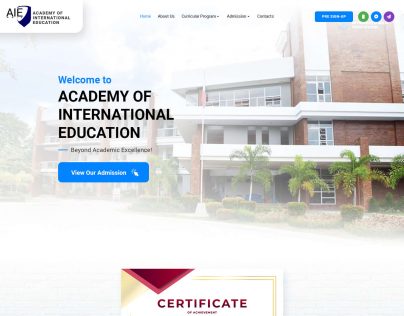This image is a screenshot of a website's homepage, featuring a muted-toned photograph in the background that depicts a red brick building, likely a school or institutional building, with three stories and palm trees in front. On the right side of the image, the front of the building is partially visible. Dominating the left side, a large headline in blue font reads "Welcome to," followed by "ACADEMY OF INTERNATIONAL EDUCATION" in bold, black capital letters. Below this headline, there is a sky-blue rectangular button with the text "View Our Admissions" in a lighter shade of blue. At the top left corner of the webpage, a logo comprising the acronym "AIE" in capital letters is displayed alongside a crescent shape and the words "Academy of International Education."